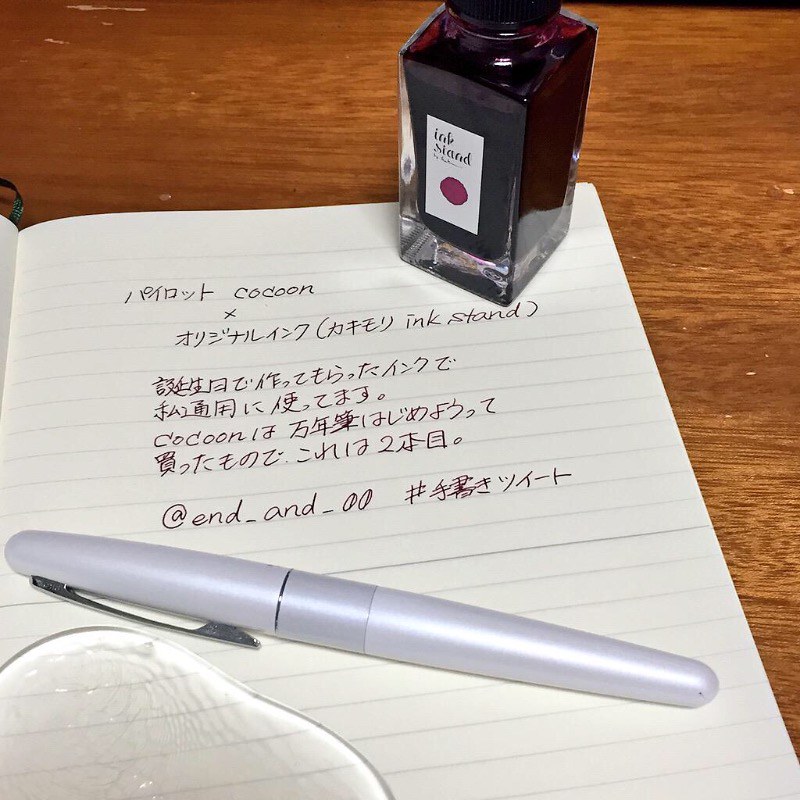This detailed photograph showcases a white, lined paper notebook with book binding, lying open on a light brown, wood grain desk. The visible part of the notebook is predominantly the right-hand page, which features several handwritten lines of text in what appears to be an East Asian language, possibly Japanese or Chinese. Interspersed among the foreign script are English words, including "cocoon" at the top line and middle of the page, and "ink stand" on the second line. Towards the bottom, the English text reads "at end_00#" followed by more non-English writing.

On the top right corner of the notebook paper rests a rectangular glass bottle filled with a dark purple substance—presumably ink. The bottle's label is a white rectangle with black text reading "ink stand," accompanied by a purple circle dot below the words, likely indicating the ink color. Additionally, a white, capped pen lies across the page, positioned near the bottom part of the photograph. Adjacent to the pen, just visible at the bottom left corner of the image, is the edge of a piece of glass.